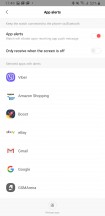This is a screenshot from a cell phone showing a blurry interface. The top section of the screen features a gray rectangle with black icons. Below that, there's some black text which is unreadable due to the blurriness. Following this, there is a gray box with more text written in a lighter gray, also not readable. The predominant part of the screen underneath displays a white background with the word "app" prominently in black, followed by smaller gray text beneath it. A noticeable small red circle is located to the right of this section.

The subsequent line is completely black, followed by a light gray rectangular strip. Below it appears to be a list, each entry accompanied by avatars. While most of the text is indecipherable, the first entry seems to start with a "V". There are seven entries in total, and the sixth one is recognizable due to the Google symbol. The fourth entry in the list possibly represents eBay. At the bottom of the screen, there is another gray box with light gray font that is too blurry to read. Overall, the screenshot is not clear enough to be legible, making it difficult to distinguish the specific content displayed.